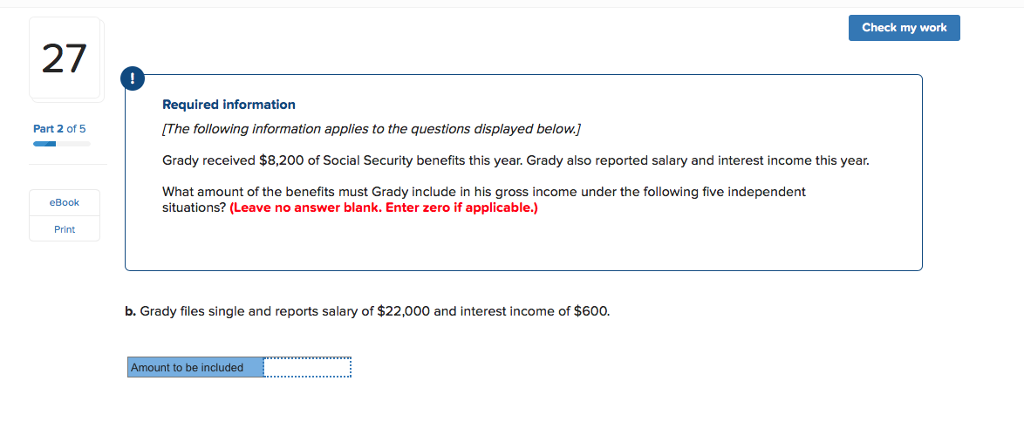### Captivating Caption for Image Description

The image appears to be a screenshot of a desktop web page, not designed for mobile devices, evident from its wide format. The page features a clean white background adorned with various interactive elements primarily formatted in blue and grey. On the left-hand side, there is a small grey-outlined square with the number "27" inside it, immediately followed by the label "part 205" in blue. Below these labels, a blue bar encompasses clickable "e-book" and "print" buttons.

In the upper right-hand corner, a blue box clearly labeled "Check my work" suggests user interactivity, likely for verifying answers or progress. Dominating the center of the screen is a white box outlined in dark blue that contains detailed informational text. At the top left of this box, a small blue circle with a white exclamation mark captures attention, indicating "required information." The supporting text beneath in black, both in and out of brackets, provides context and instructions for the displayed question.

The scenario outlines that Grady received $8,200 in social security benefits and additional salary and interest income. Users are prompted to determine the amount of benefits to include in Grady's gross income under five independent situations. Specific instructions are highlighted in red text: "Leave no answer blank, enter zero if applicable."

Immediately below this, a sample question states: "Grady filed a single report salary of $22,000 and interest income of $600," followed by an interactive bar where users input the "amount to be included" in black text. The bar transitions from shaded blue to a blue dotted outline, suggesting an input mechanism, possibly for an online exam or financial calculation tool.

The highly detailed, structured layout and color coding support user navigation and input within an online testing environment, likely dealing with tax calculations or financial training.